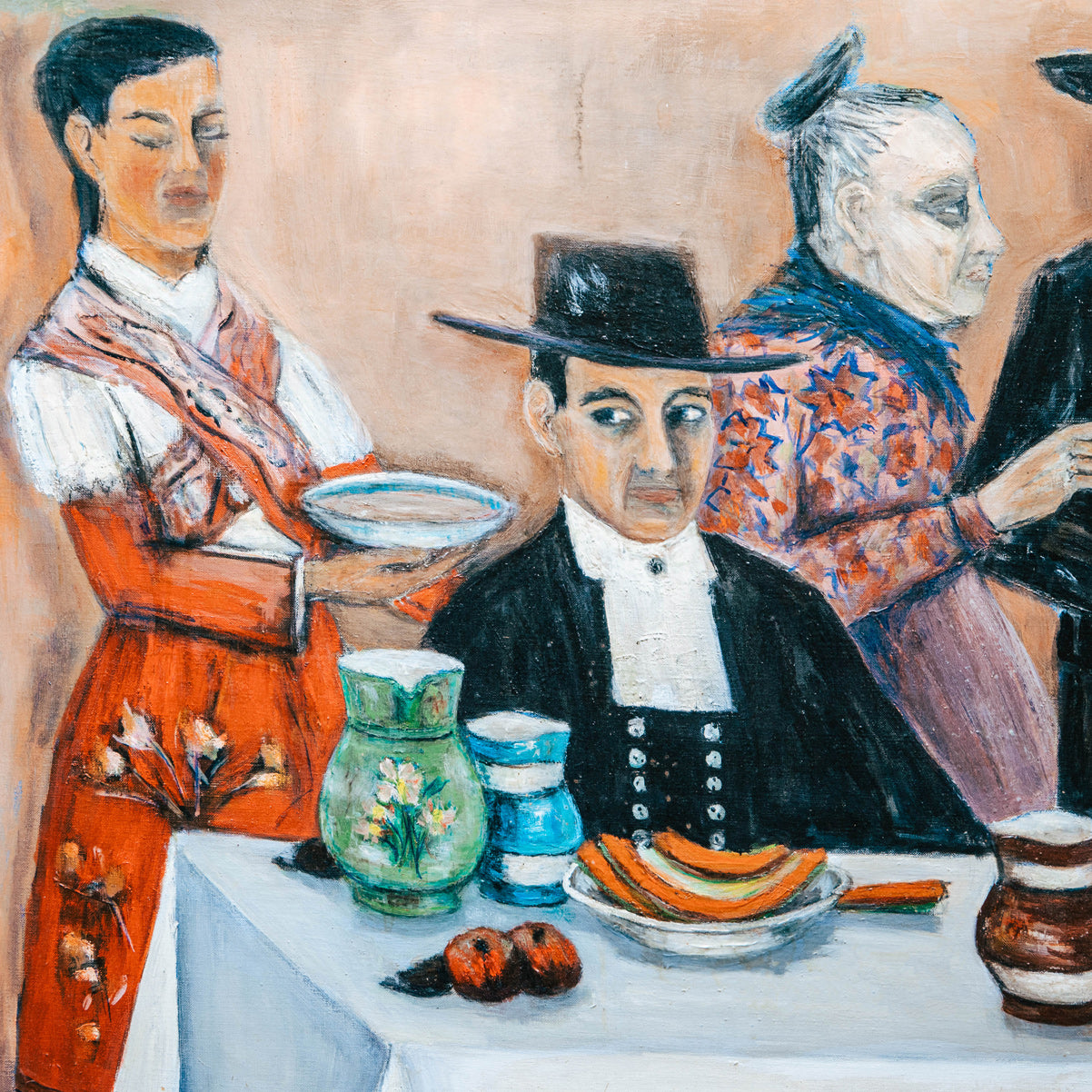This vibrant, Mexican-style painting, possibly by a female artist associated with Leon Trotsky, depicts a colorful, somewhat cartoonish scene. At the center, a man in formal traditional Mexican attire—a black tuxedo-like suit and a black cowboy hat—sits at a table with a white tablecloth. His eyes dart to his right, observing a woman with brown hair dressed in an orange top and pants, adorned with a floral pattern, who appears to be serving him soup. The table is adorned with various foods: two red apples, a white dish with orange, rind-like shapes, a green pitcher with flowers, and a blue and white mug. To the man's left, an older woman in a detailed dress featuring flowers or stars, with her gray hair tied back, gazes off to the right. Partially visible on the far left, another figure in black sleeves completes the composition. The background features additional ornate elements, such as a blue table and possibly a serving vessel, enhancing the overall rich and detailed narrative of the painting.